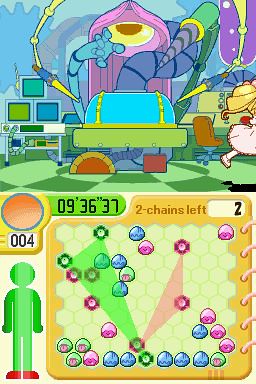This image is a vibrant screenshot of a cartoon-style phone or computer game. The colorful top half showcases a green checkered floor surrounded by an array of machinery and computers positioned on the left side. A robotic hand, also bright blue, reaches over a tank of the same vivid hue amidst the lively backdrop filled with varied hues of purple, pink, yellow, and green tools scattered around.

The bottom half features a detailed map or diagram peppered with different colored circles. To the map's left stands a green stick figure sporting red shoes, with the number "004" displayed above it. In a box containing the map, there is a text indicating "Two chains left," accompanied by numbers "936" and "37" neatly placed to the left.